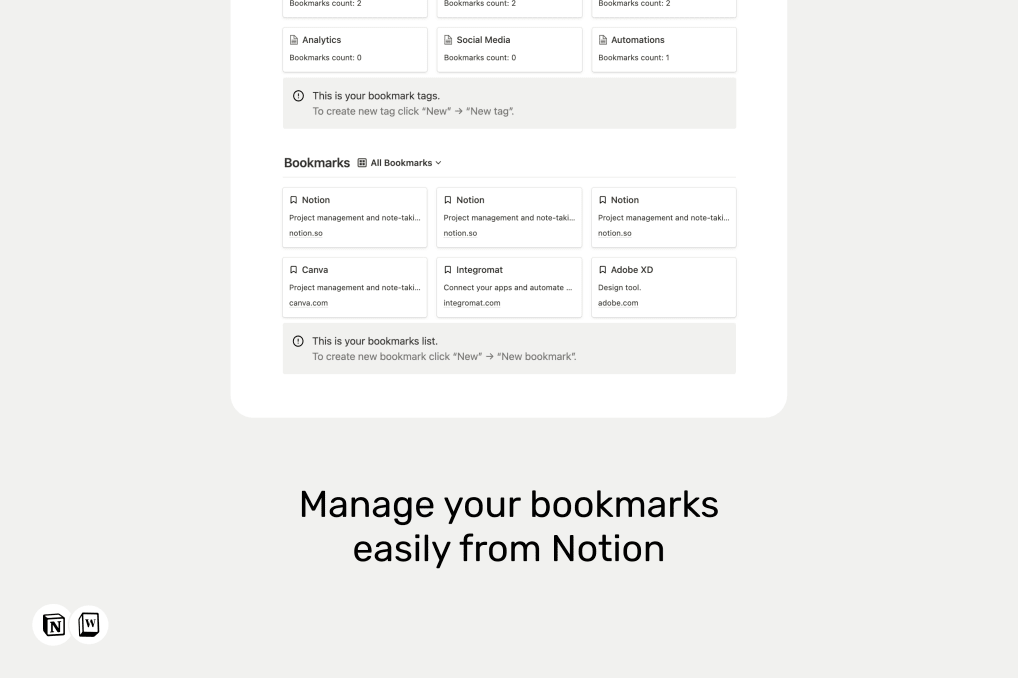This image showcases a user interface for managing bookmarks within Notion. The bottom of the image features the text "Manage your bookmarks easily from Notion." At the top of the image, there is a white page with a grid layout consisting of 3 columns and 4 rows. 

The first row appears to have some obscured text but indicates "Bookmark count: 2" followed by "Analytics, bookmarks count: 0." Below this is the visible section labeled "Bookmarks," with an adjacent section labeled "All Bookmarks."

In the "Bookmarks" section, there are multiple blocks: the first three blocks are labeled "Notion," likely representing specific bookmarks within Notion that bear similar content. The subsequent blocks are labeled "Canva," "Integrament," and "Adobe XD," suggesting a variety of external bookmarks managed through the interface.

This layout provides an organizational tool for users to efficiently manage and access their bookmarks in Notion.